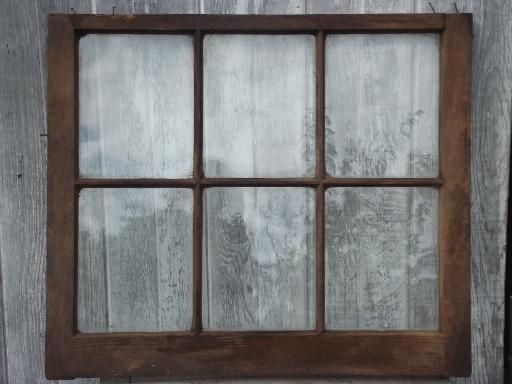This grainy color photograph is a closeup of an older, textured wooden window frame with a dark brown to light brown hue. The window, which seems more decorative than functional, has six rectangular panes arranged in three columns and two rows. Each pane is separated by the wooden framework and partially obscured by reflections on the glass. These reflections suggest a scenic backdrop that includes trees and possibly mountains, giving the impression of a picturesque setting seen during the evening or on a cloudy day. The glass reflects the light, adding a sense of depth to the image. The window appears to be affixed to a gray, textured wooden fence or door, with nails visible around its edges, securing it in place. The overall atmosphere of the photo is somewhat gloomy, dominated by dark and muted shades of brown and gray.